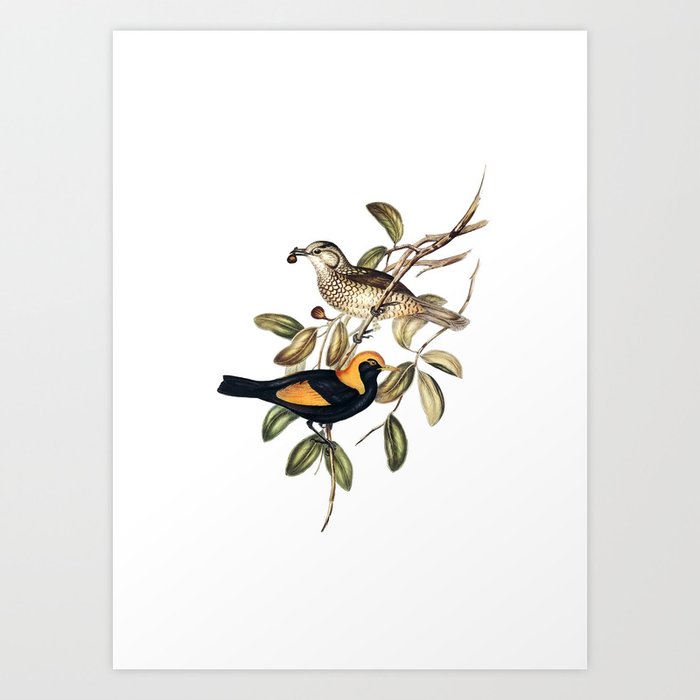This image portrays a detailed drawing of two birds perched on tree branches, set against a stark white background. The branches, extending diagonally from the right with some splitting off to the left, feature vibrant green leaves that are oval-shaped, some with central splits and others showing a hint of turning brown. The bird situated lower on the branches is black with striking orange on its head and wings, complemented by a sharp, yellow beak and tail feathers. Above it, facing in the opposite direction, is a bird characterized by a tan, white, and gray plumage, holding a small seed or nut in its beak. The artist's strokes vividly capture the textures and intricate details of the birds' feathers, the leaves' veins, and the lifelike portrayal of the scene, set on paper against a simplistic blue background, adding depth and contrast to this nature-inspired artwork.